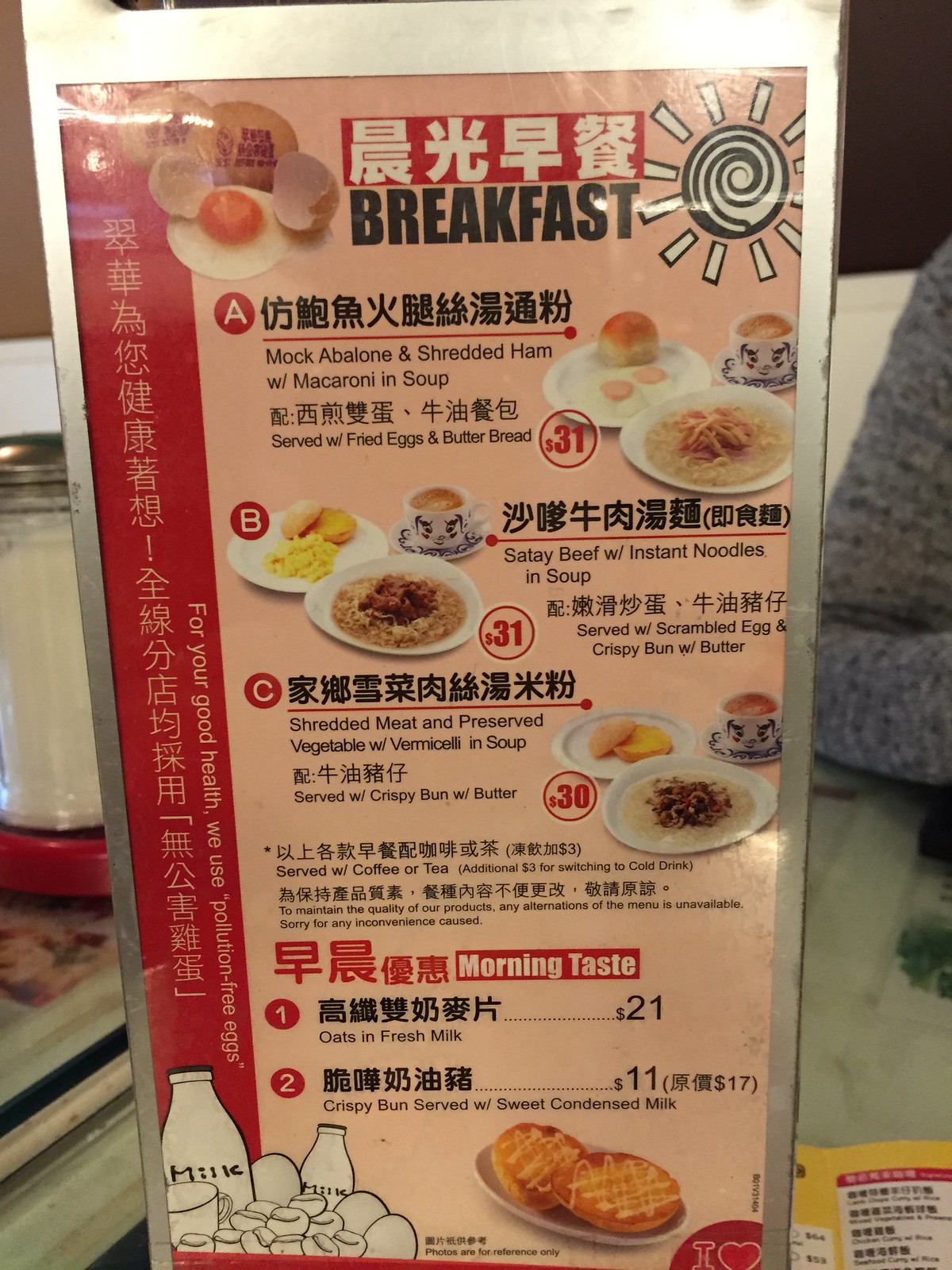A laminated menu, detailed in a mix of English and Chinese characters, stands vertically with a glossy surface reflecting light. It is framed in a thin metal holder. In the background to the right, an arm clad in a gray sweater holds a white tote bag and a smaller yellow menu. To the left, a large salt or sugar shaker with a silver top rests on a counter. The menu features a light peach background with a red strip running down the left side. The word "Breakfast" along with Chinese characters is displayed at the top. An artistic black-and-white sun with a spiral center adorns the upper right corner, while the upper left corner showcases a graphic of two whole eggs and one fried egg. The upper portion of the menu lists three prominently bolded breakfast items, each accompanied by a photograph depicting two plates of food and a cup of tea. The lower section presents two more items, depicted alongside an image of a pastry. A black-and-white drawing of milk and eggs is situated in the lower left corner.